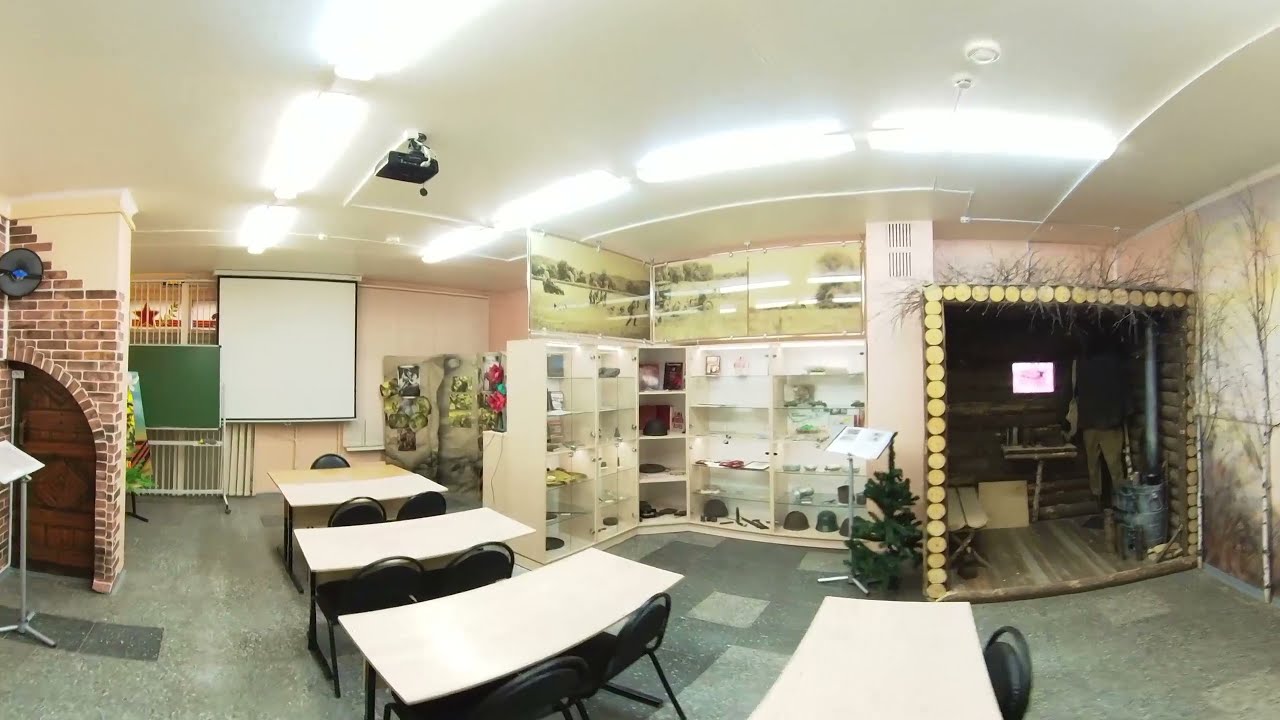This panoramic image depicts a spacious, eclectic classroom characterized by its varied color palette and diverse furnishings. The walls exhibit a mix of white, salmon, red, green, yellow, and brown hues, creating a lively environment. The gray tile or linoleum floor anchors the room's elements. 

Centrally positioned are several tables with white laminate tops, each accompanied by two black chairs. These are primarily located on the bottom left side of the image, suggesting a focus area for group activities. Above this cluster of tables, a projector screen hangs from the ceiling, shaded by recessed fluorescent lights illuminating the room's varied zones.

On the far right, there is a unique small hut-like structure composed of different types of wood, seemingly designed for breakout activities or isolated study. Adjacent to it is a display case filled with assorted items. Against the back wall are open bookshelves with multiple rows of cubby-like divisions, storing books, mats, and other educational supplies, hinting at its use by schoolchildren.

To the left side, there is a portable chalkboard on wheels that complements the wall-mounted green chalkboard and a whiteboard. These diverse instructional tools face the rows of tables. A distinctive feature on the leftmost wall is a partition with a graphic of a brick facade and a wooden arched door, potentially serving as a whimsical educational decor. 

The overall vibrant and multifaceted setup, inclusive of modern technology like the ceiling-mounted projector and practical storage solutions, underscores the room’s function as a dynamic learning space.